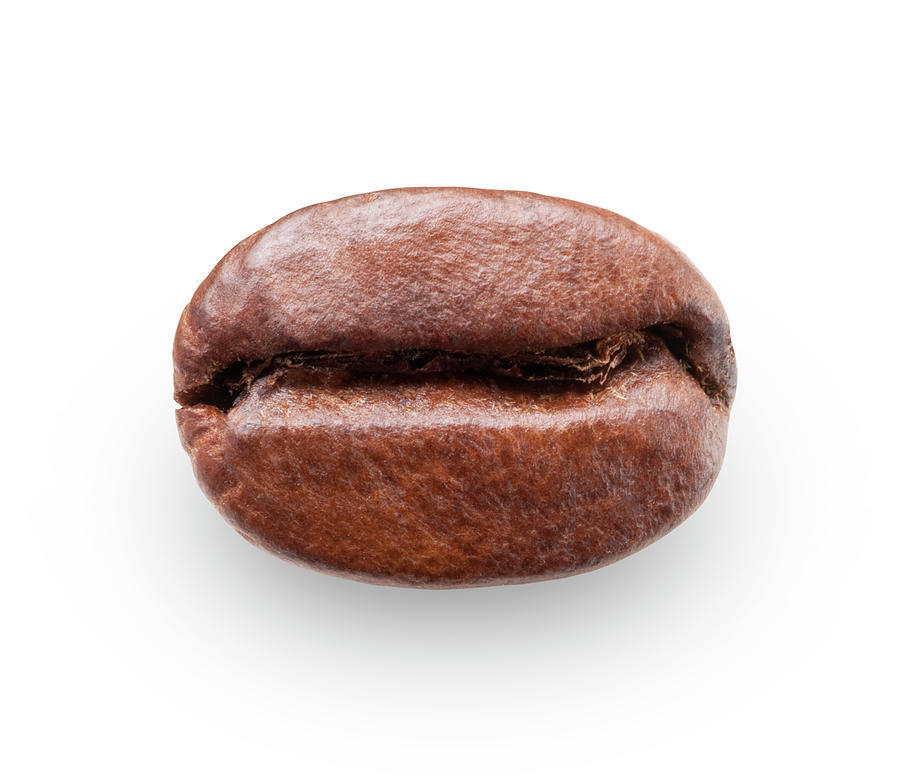This close-up image features a single dried coffee bean centered against a stark white background. The bean is an elongated oval shape with a prominent, dark ridge running lengthwise through its center, creating a deep shadowed indentation that highlights its textured surface. The bean's glossy surface displays small irregularities and indicates a slightly oily texture. The rich coloration of the bean varies from dark brown to lighter brown hues, with subtle reddish tints interspersed throughout. The drop shadow beneath the lower half of the bean adds depth to the image, accentuating its three-dimensional form. This detailed and vibrant depiction could serve as a promotional photograph, showcasing the characteristic qualities of a typical medium roast coffee bean.